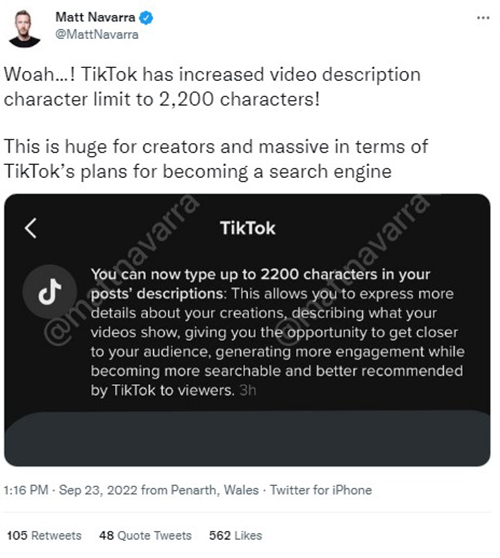**Detailed Caption:**

This vertically oriented image captures a screenshot of a tweet from Twitter. The background is the typical white interface of a computer screen. In the upper left-hand corner, there is a profile picture of the user Matt Navarra. Next to the profile picture, you see the name "Matt Navarra" accompanied by a blue verification checkmark and the Twitter handle "@MattNavarra." On the upper right-hand side of the image, there are three horizontal gray dots indicating options.

The content of the tweet itself is highly informative and exciting for content creators. It reads: "Whoa...! TikTok has increased video description character limit to 2,200 characters. This is huge for creators and massive in terms of TikTok's plans for becoming a search engine."

Below the tweet, there is a black rounded horizontal rectangle with a music icon and the word "TikTok." The text within this rectangle elaborates on the update: "Matt Navarra, you can now type up to 2,200 characters in your post descriptions. This allows you to express more details about your creations, describe what your videos show, and give you an opportunity to get closer to your audience, generating more engagement while becoming more searchable and better recommended by TikTok viewers."

The timestamp at the bottom of the tweet indicates that it was posted three hours ago at 1:16 PM on September 23, 2022, from Penarth, Wales via Twitter for iPhone. The tweet also displays metrics showing the number of retweets, quote tweets, and likes it has received.